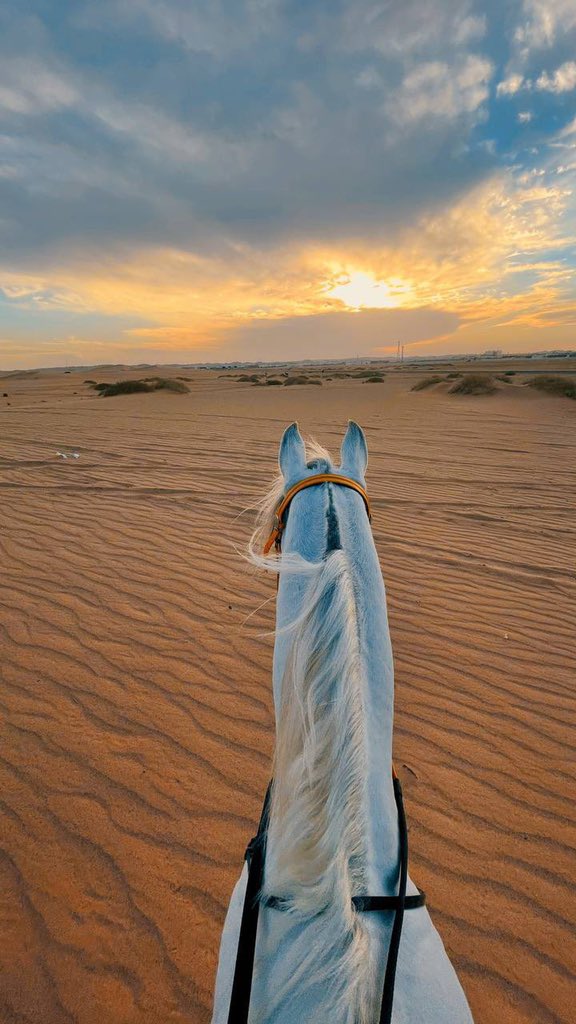The color photograph captures the point of view from someone riding a white horse in a vast desert landscape. The horse's neck and head dominate the center of the frame, highlighting its white mane with a silvery-blue tint. Black reins are draped around the horse's neck, and a tan strap is visible under its face and behind its ears. The sandy terrain stretches endlessly with occasional small dunes and dry, cut bushes scattered in the foreground. In the far distance, a few small buildings and hills can be seen. The sky is intermittently cloudy with hues of yellow and blue, suggesting either sunrise or sunset, with the sun partially obscured by clouds. The photograph is taller than it is wide and shows no other people or animals.